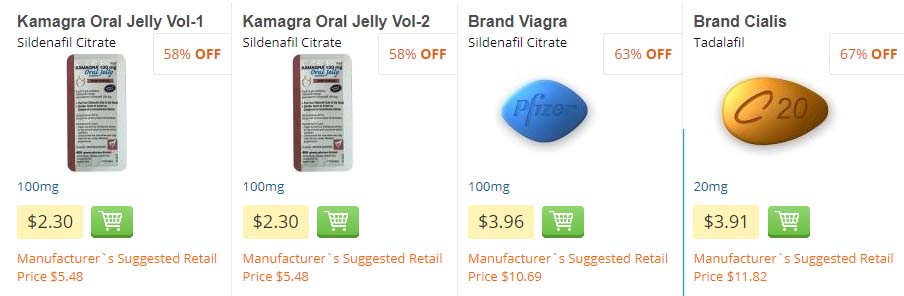The image showcases four products for sale, each with a detailed visual and discount information. From left to right, the products are:

1. **Comagra Oral Jelly Vol-1**: Packaged product with a 58% discount (indicated in red text). Priced at $2.30, down from the manufacturer's suggested retail price of $5.48.
2. **Comagra Oral Jelly Vol-2**: Packaged product with a 58% discount (indicated in red text). Priced at $2.30, down from the manufacturer's suggested retail price of $5.48.
3. **Brand Viagra**: Displayed as a blue pill with a 63% discount. Priced at $3.96, down from the manufacturer's suggested retail price of $10.69.
4. **Brand Cialis**: Displayed as a gold pill with a 67% discount. Priced at $3.91, down from the manufacturer's suggested retail price of $11.82.

Each product is highlighted with a diagram beneath it, showcasing the packaging for the first two items and the pill form for the last two. The dosage information is included in blue text, with all products at 100 milligrams except for Brand Cialis, which is at 20 milligrams. The background of the image is white.